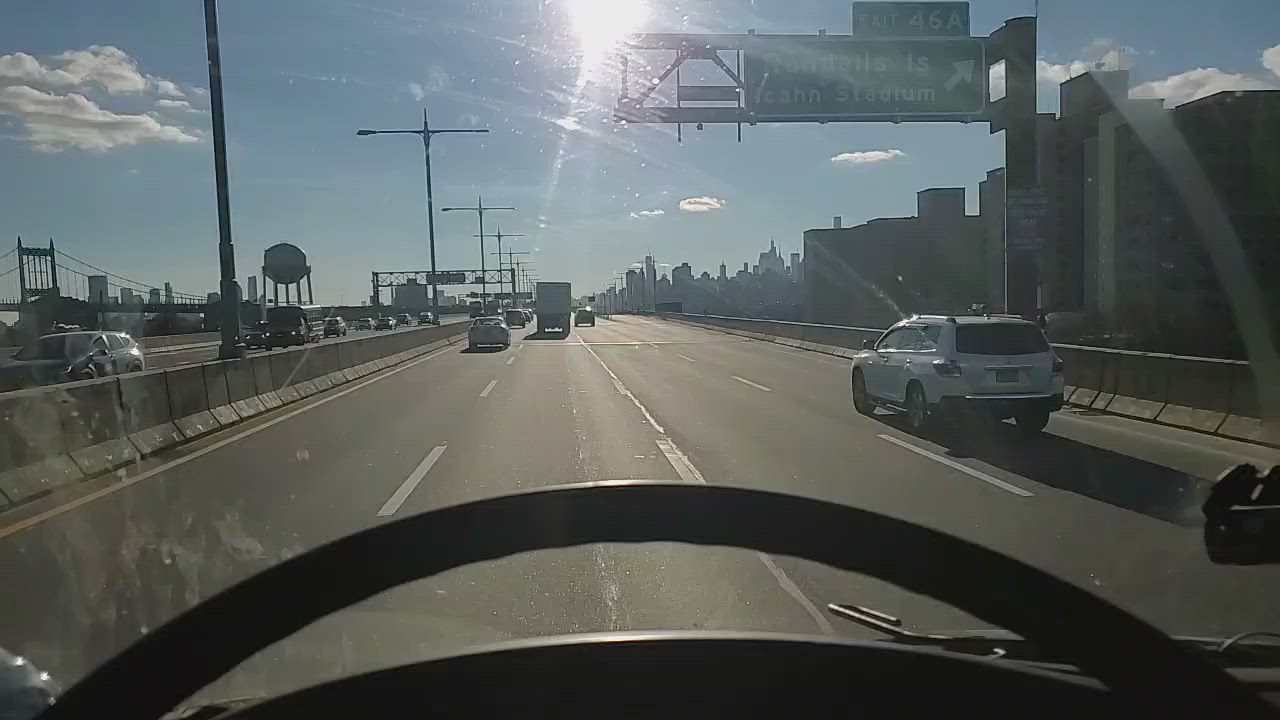A high-angle photograph taken from within a large vehicle captures the view through its clear windshield. Visible from the driver's perspective, the steering wheel partially frames the image. To the right, a white van can be seen on the road. In the distance, an urban skyline composed of several tall buildings stretches across the horizon under a vibrant blue sky dotted with fluffy white clouds. Central to the composition is a green traffic sign that reads "Exit 46A. South of the Stadium." Various light poles line the middle of the scene, their lights extending forward along the street. Further into the background, a substantial water tank with structural supports and a distant bridge add additional layers to the urban landscape.